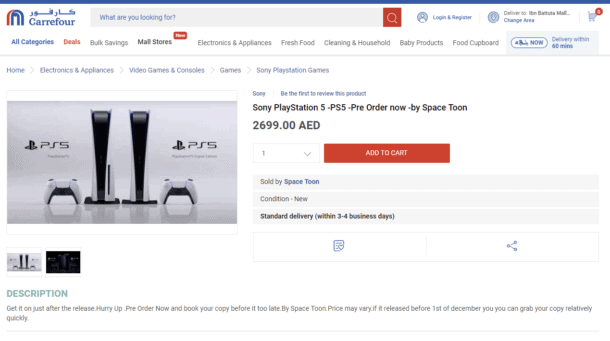This screenshot from Carrefour's website showcases their online shopping interface, elegantly organized for ease of use. At the top, a dark blue navigation bar includes essential user tools: a search box with the prompt "What are you looking for?" accompanied by a red magnifying glass icon, login and register buttons, a "Deliver to" area adjustment option, and a shopping cart icon. 

Beneath this, various tabs provide quick access to different categories: All Categories, Deals, Bulk Savings, Mall Stores, Electronics & Appliances, Fresh Food, Cleaning & Household, Baby Products, Food Cupboard, and a highlighted light blue rectangle indicating a "Delivery within 60 minutes" service.

The main focus of the screenshot is on a product listing for the Sony PlayStation 5 (PS5). The breadcrumb navigation shows the product’s categorization: Home > Electronics & Appliances > Video Games & Consoles > Games > Sony PlayStation. The central image is predominantly grey with two PS5 consoles and two controllers, captioned "PS5."

Next to the image, the product details are clearly displayed: "Sony PlayStation 5, PS5," priced at 2,699 AED, sold by Spacetune. The delivery time is estimated at three to four business days. Consumers can select the quantity and add the item to their cart with an easily accessible button. 

Underneath the main image are two thumbnail images for additional views of the product. A descriptive section beneath these images urges customers to pre-order to secure their PS5 before the official release date, noting that prices may vary if the product is released before December 1st. It highlights the urgency and the opportunity to receive the console shortly after release.